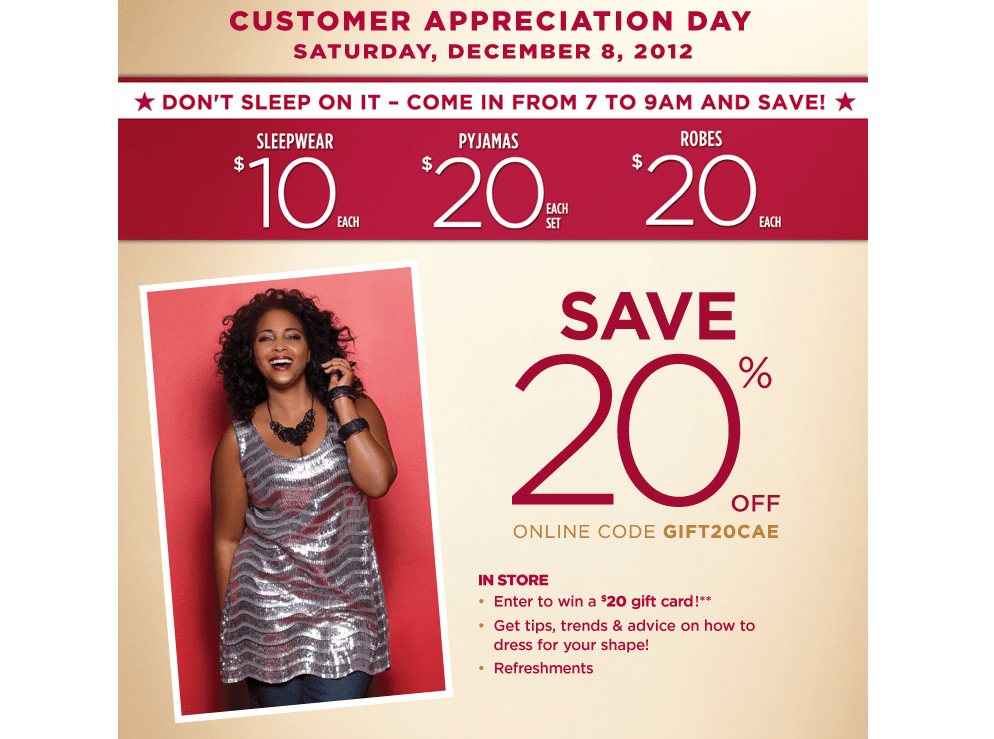**Customer Appreciation Day Advertisement (Square Frame)**

The advertisement features a tan background that subtly fades to a lighter tan towards the center, creating a warm and inviting ambiance. Prominently displayed at the top, in bold red uppercase letters, is the event announcement: "CUSTOMER APPRECIATION DAY, SATURDAY, DECEMBER 8, 2012."

Just below this announcement, a narrow horizontal white banner accented with a red top edge urges customers not to miss out: "Don't sleep on it, come in from 7 to 9 a.m. and save."

Descending further, a slightly taller horizontal red banner highlights special offers in white text:
- **Sleepwear: $10 each**
- **Pajamas: $20 per set**
- **Robes: $20 each**

On the left side of the frame, there's an image of a woman smiling radiantly. She accessorizes her shimmery silver tank top with a black necklace and two black bracelets on her left arm, which is bent and extended towards her face while her right arm rests behind her.

To the right of the image, the ad continues with more savings: "Save 20% off online with code GIFT20CAE." Additionally, it entices customers to visit the store to enter a raffle for a $20 gift card, along with an opportunity to receive tips, trends, and advice on how to dress for their shape, all while enjoying refreshments.